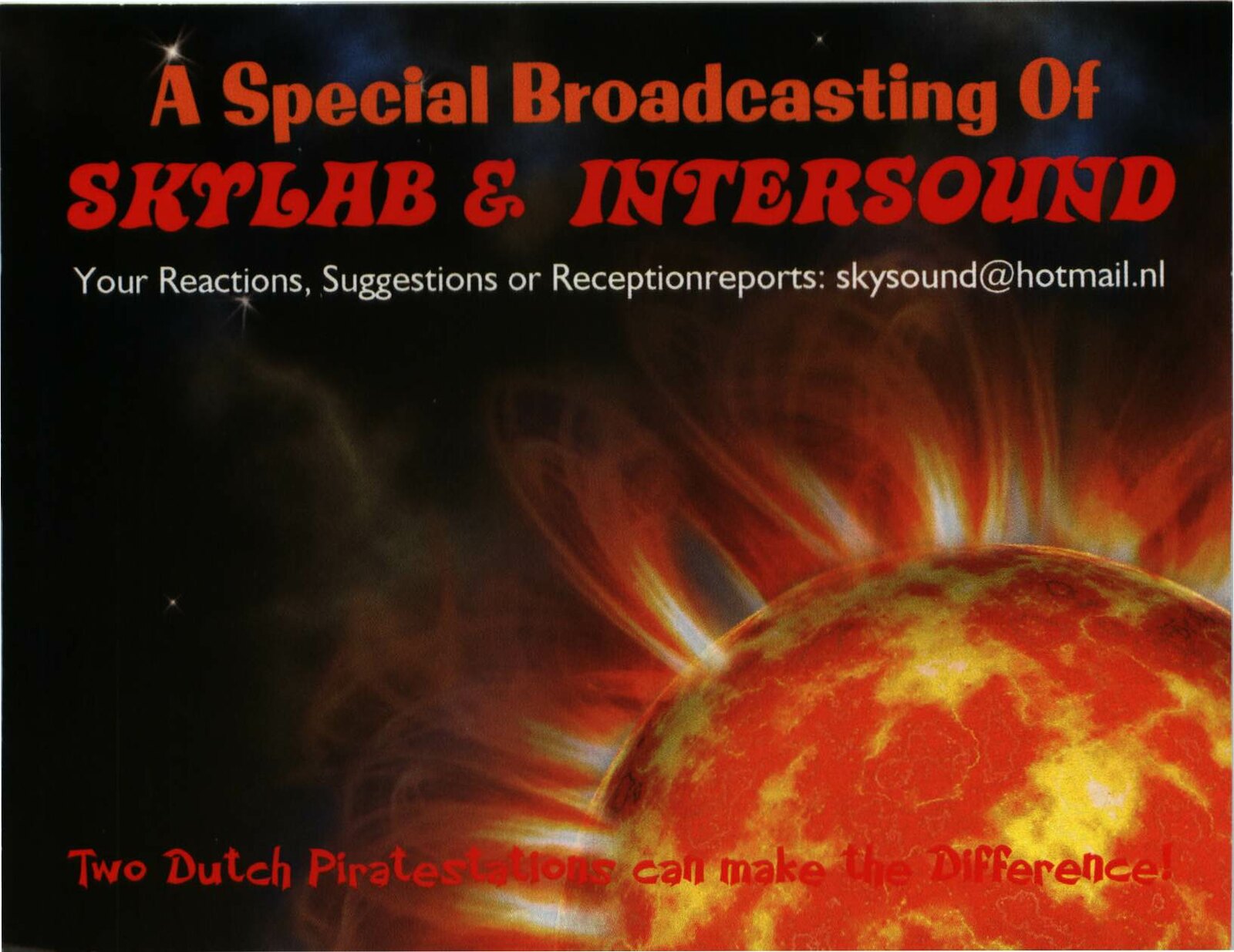This vibrant and visually intense image features a dramatic depiction of a large red and gold planet, possibly the sun, against a black background. Solar flares or fiery explosions in shades of yellow, orange, and red burst outward into the dark expanse of space, conveying intense heat and energy. At the top of the image, bold red letters announce "A Special Broadcasting of Skylab and Intersound," while smaller white text beneath invites viewer engagement: "Your reactions, suggestions, or reception reports: skysound@hotmail.nl." At the bottom, in red letters, the image concludes with the phrase, "Two Dutch pirate stations can make the difference." The combination of fiery celestial activity and striking text creates an eye-catching and evocative advertisement.